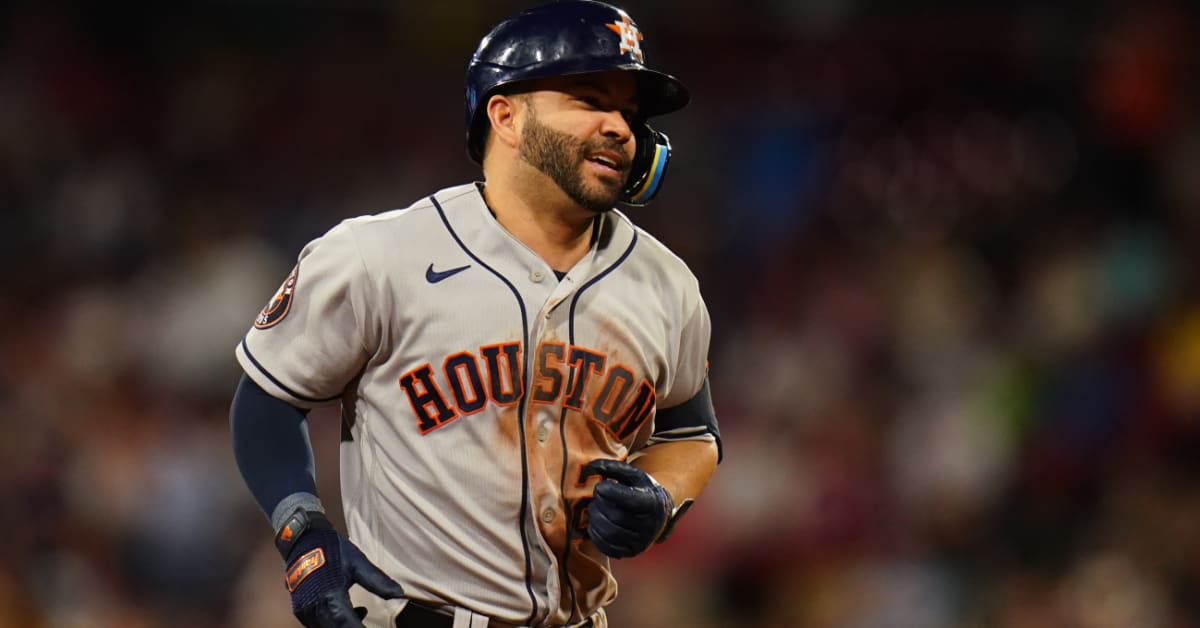A Houston baseball player is depicted, showcasing a celebratory expression, likely after a successful play. He is adorned in a light gray shirt prominently featuring the word "Houston" in substantial black lettering, accented by a thick orange outline that makes it stand out. Complementing his attire, he sports a pair of tight, long dark blue sleeves and matching dark blue gloves. His hard hat is dark blue, emblazoned with a star emblem at the front. The player's equipment includes a black device with a blue and yellow stripe, possibly an earpiece, visible on the left side of his face as he looks to the right. In the background, the indistinct and blurred crowd adds a dynamic backdrop, consisting primarily of white and various colored shapes. The player's joyful demeanor encapsulates the spirit of the moment, adding to the overall lively atmosphere of the scene.